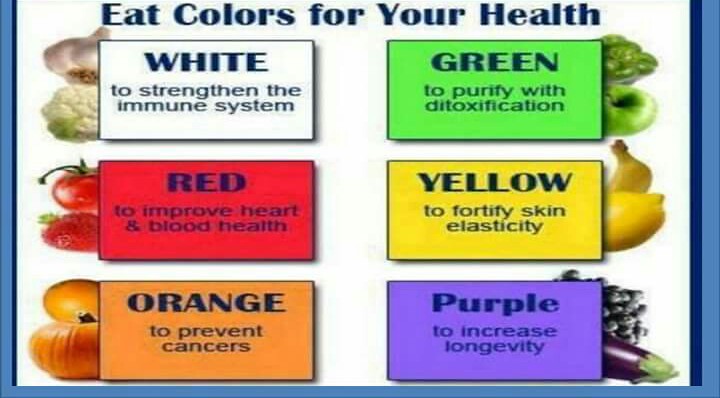The image features a flyer with a blue border and a white background. At the top, it emphasizes in blue letters, "Eat Colors for Your Health." The flyer is divided into several colored sections, each accompanied by corresponding fruits or vegetables and a health benefit.

- The first section is a white box with blue letters that say "White to strengthen the immune system," accompanied by images of garlic and cauliflower.
- Below it, a red box with black letters states "Red to improve heart and blood health," featuring pictures of a tomato and a strawberry.
- Next, an orange box with black letters reads "Orange to prevent cancer," displaying a pumpkin and an orange.
- On the right side, there are additional colored boxes:
  - A green box claims "Green to purify with detoxification," with images of an apple and another green fruit.
  - A yellow box says "Yellow to fortify skin elasticity," with images of a lemon and a banana.
  - A purple box states "Purple to increase longevity," featuring an eggplant and blueberries.

The flyer suggests incorporating a variety of colored foods into your diet to boost different aspects of health, visually presenting each color-coded health benefit alongside a corresponding fruit or vegetable.